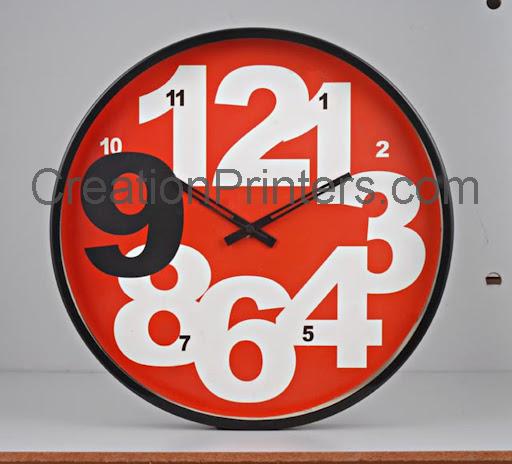This photograph depicts a striking clock with a bold red face, likely designed for an advertisement typically seen in magazines. The clock prominently features large numerals for 12, 1, 3, 4, 6, 8, and 9, with the latter being black while the rest are white. Smaller numerals, 10, 11, 2, 5, and 7, are scattered within these larger numbers; 10 and 2 are white, while 11, 1, 5, and 7 are black. It has both minute and hour hands. The image includes a watermark that reads "creationprinters.com." The clock appears to be placed on a white shelf or bookcase, with a brown strip, likely part of the shelf, visible at the bottom. Two indistinct black marks can be seen on the right side of the image, though their exact purpose is unclear—they could be part of the watermark or the shelf. The clean, minimalist background emphasizes the vibrant, eye-catching design of the clock.